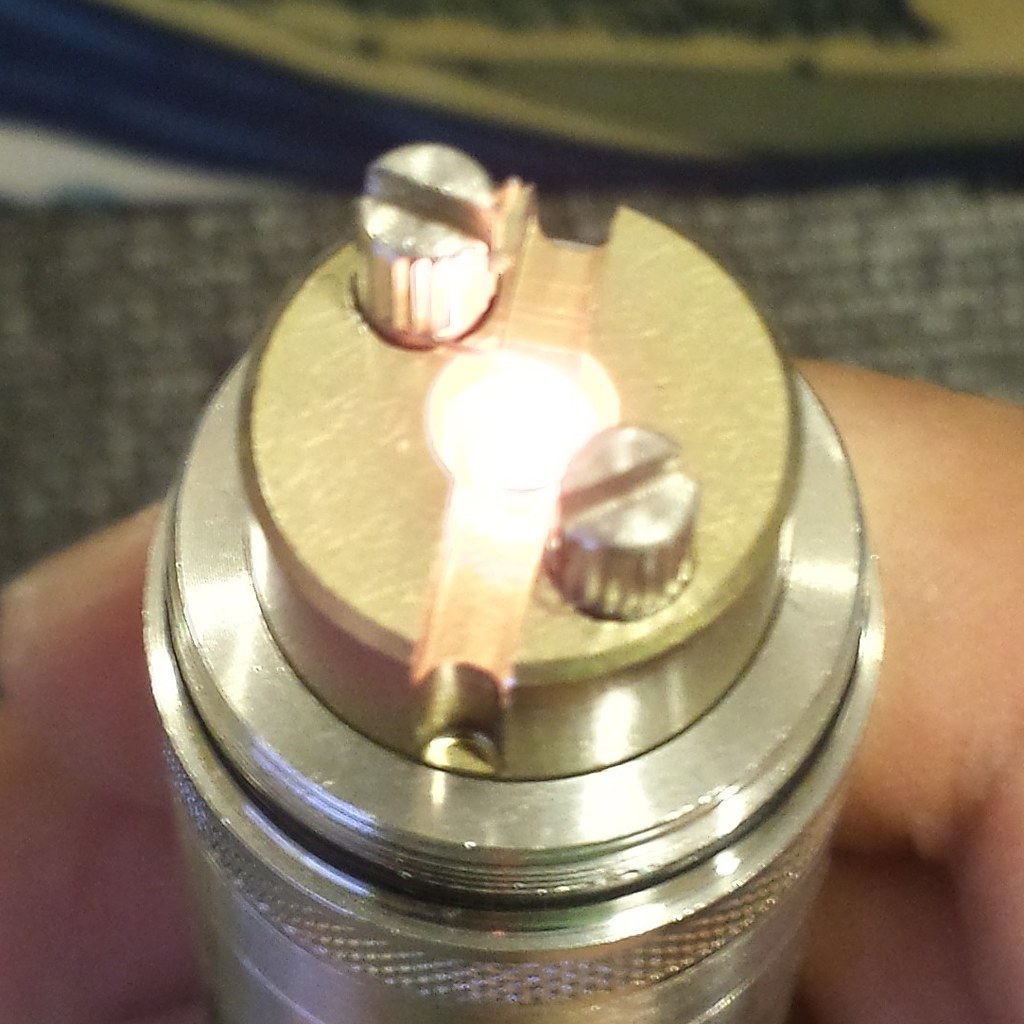The image is an up-close, albeit blurry, shot focusing on an intricate object being held by a person's hand. The object appears to be metallic with a series of cylindrical components. It has a larger silver cylinder at the base, which houses two smaller, concentric cylinders that diminish in size as they ascend. The smallest cylinder at the top is gold-ish in color and features a groove down the center reminiscent of a flathead screw. This grooved cylinder also has light reflecting off its top, creating an illuminated, circular effect. 

On either side of this gold cylinder, positioned diagonally from one another, are two additional smaller cylindrical protrusions with similar grooves. These resemble screws and are also highlighted by the light, giving a detailed view of their ridged sides. In the background, there are hints of a yellow and dark blue layer, alongside a textured gray area that might be a table placemat or rug. Overall, the shot captures the complex, layered design of this metal object, possibly a plug or torch-like tool, with a distinct interplay of silver and gold elements.